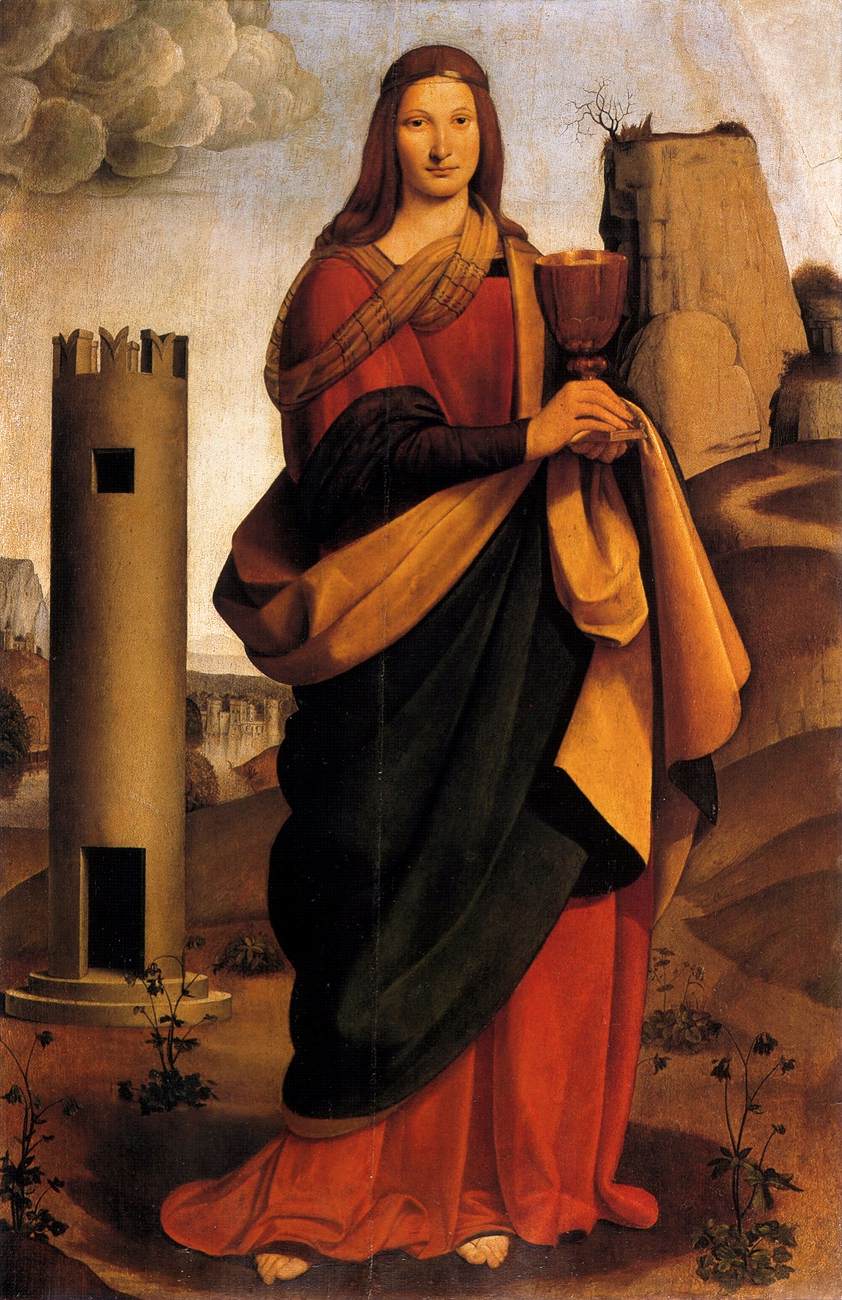This is a detailed painting set in the olden days, likely during the Renaissance or Elizabethan times, depicting a woman standing outside. She is dressed in a layered outfit with a striking red robe, a black cloak that reveals a gold lining, and a scarf around her neck. Her long hair, a mix of red and brown tones, flows down her back. The woman stands on sandy, hilly terrain, perhaps a dirt path, with a prominent stone castle tower to her left and rocky formations to her right—these rocks may also be part of the castle structure. The background shows a landscape of rolling hills and plateaus, with more castle structures faintly visible in the distance. She holds a chalice or goblet in front of her, adding an element of intrigue. Above her, the sky is clouded, casting a somewhat somber, dark tone over the scene, though the beige hues of the landscape are punctuated by the vivid red of her robe.